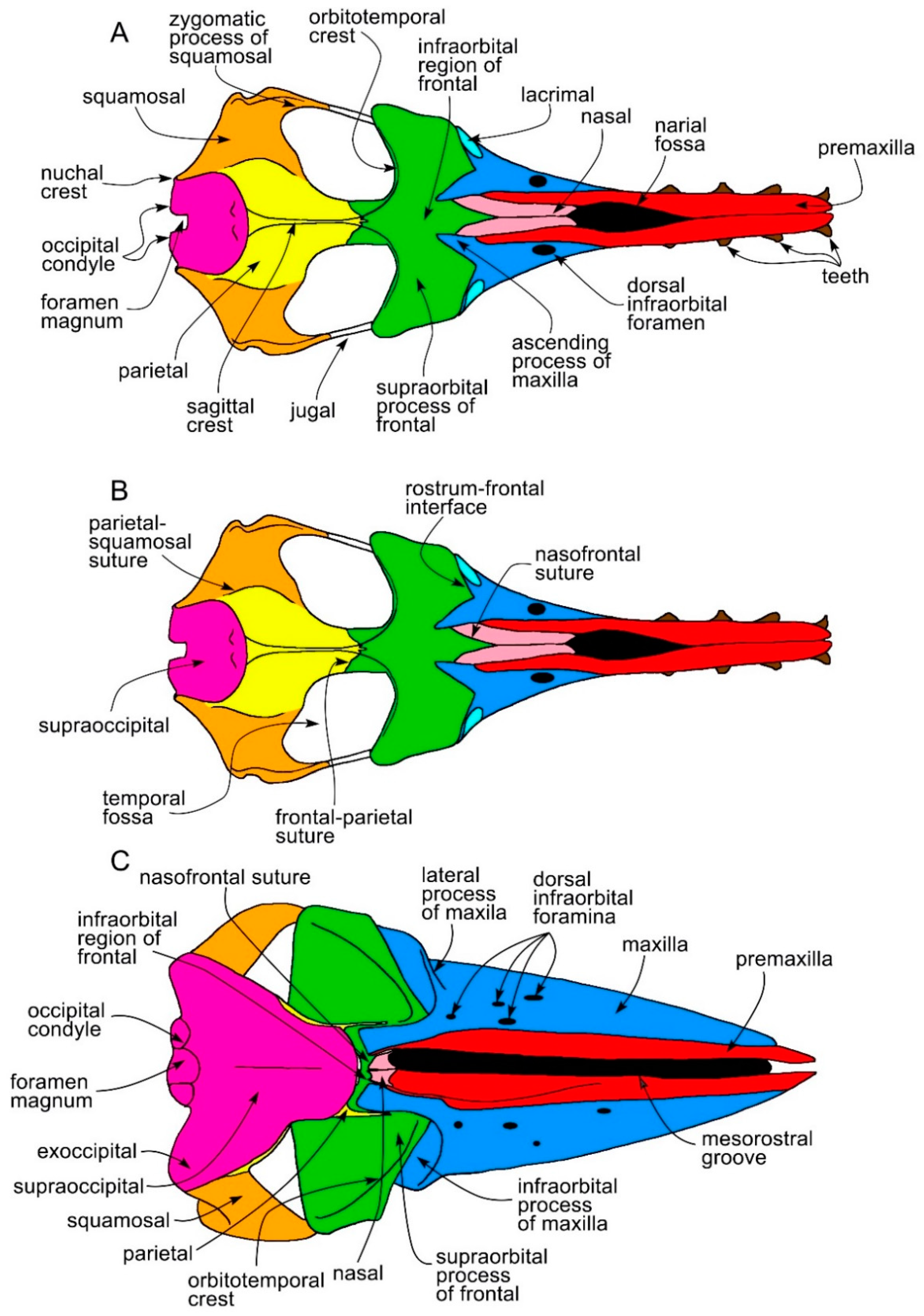The image features three highly detailed, colorful diagrams arranged vertically, labeled A, B, and C, showcasing the dorsal views of a dolphin's skull. Each diagram meticulously illustrates various anatomical parts, highlighted in vibrant colors such as pink, orange, yellow, green, blue, and red. Key components like the zygomatic process of the squamosal, orbitotemporal crest, lacrimal, nasal, premaxilla, dorsal tooth row, and infraorbital foramen are clearly labeled. The structure and layout of the bones, with different sections demarcated in distinct colors, provide an insightful look into the complex cranial architecture, suggesting a scientific illustration aimed at detailed anatomical study.